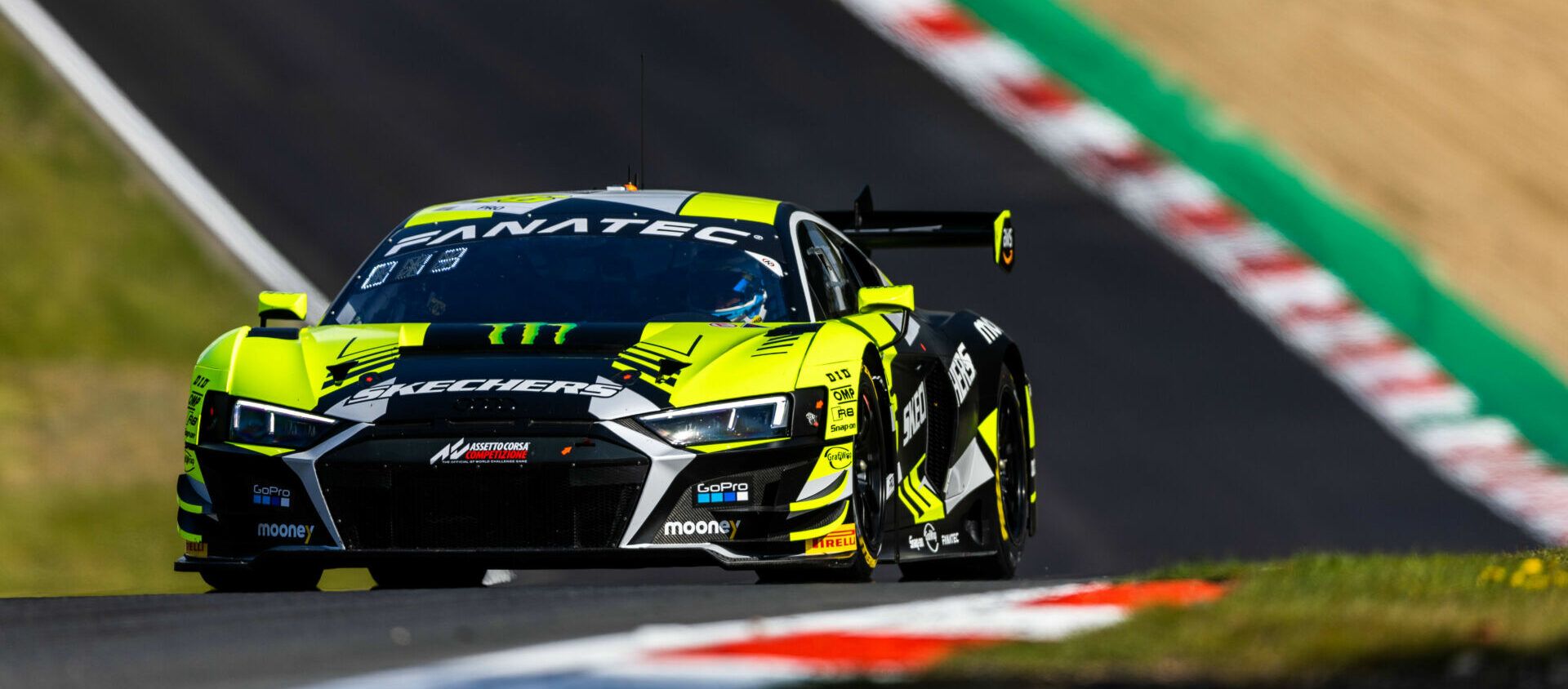This is a detailed, horizontal photograph of a vibrant race car on a race track. The image is mostly focused on the car itself, captured from a low, three-quarter front angle, giving the sense that the photographer is almost laying on the ground. The racetrack features a striking combination of green, red, and white markings atop black pavement, flanked by lush green grass. The track appears to ascend uphill to the left in the background, lending a dynamic sense of movement. The race car is a hot rod sedan in a striking yellow with black highlights, accented by a red stripe and multiple logos. The windshield prominently displays the word "FANATIC" in bold letters, with "013" beneath it in white. The hood also features "SKETCHERS" and the logos "ACID," "ACETO CORSA COMPLECIONE," while the lower left and right fenders show "GOPRO" and "MOONIE." The front end includes a Monster logo, adding to its distinctive appearance. The car is captured in motion, driving forward, and framed against the contrasting green and black background of the track.